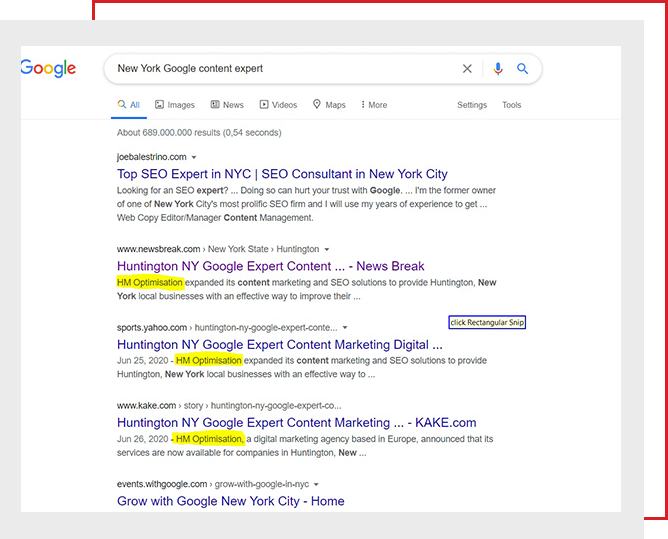The image depicts a web browser page with a search query related to top CEOs and Google content experts in New York City. The search bar shows the query "New York Google Content Expert," returning around 689 million results. The top result reads, "Top CEO Expert in New York City, SEO Consultant in New York City." Another notable result from cake.com highlights, "Huntington, New York, Google Expert, Content Marketing." Additionally, H&M Optimization, a digital marketing agency based in Europe, has announced that its services are now available for companies in Huntington, New York. Websites listed include JoeBallestrino.com, newsbreak.com, sports.yahoo.com, and eventswithgoogle.com, as well as Grow with Google New York City Home.